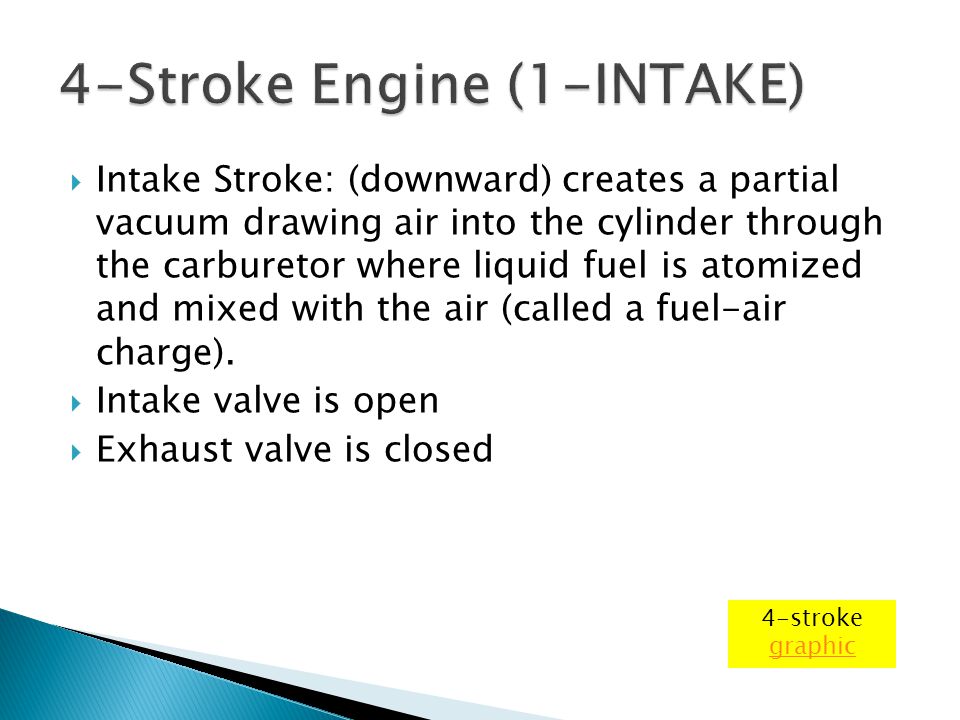The image depicts a PowerPoint-style presentation screen titled "Four-Stroke Engine (1-Intake)" in large black text within a yellow box, featuring a clickable red link labeled "graphic." Below the title, there is a detailed description of the intake phase of a four-stroke engine, explained through three blue, right-pointing triangular bullet points. The first bullet highlights the "intake stroke" where a downward motion creates a partial vacuum, drawing air into the cylinder through the carburetor, atomizing and mixing liquid fuel with the air (referred to as a "fuel-air charge"). The second bullet states "intake valve is open," and the third bullet explains "exhaust valve is closed." The visual also includes a series of overlapping triangles in blue, black, and gray at the lower left corner, adding a stylish, yet unclear visual element. The overall presentation is very textual and informative, emphasizing the mechanics of the engine's intake process.